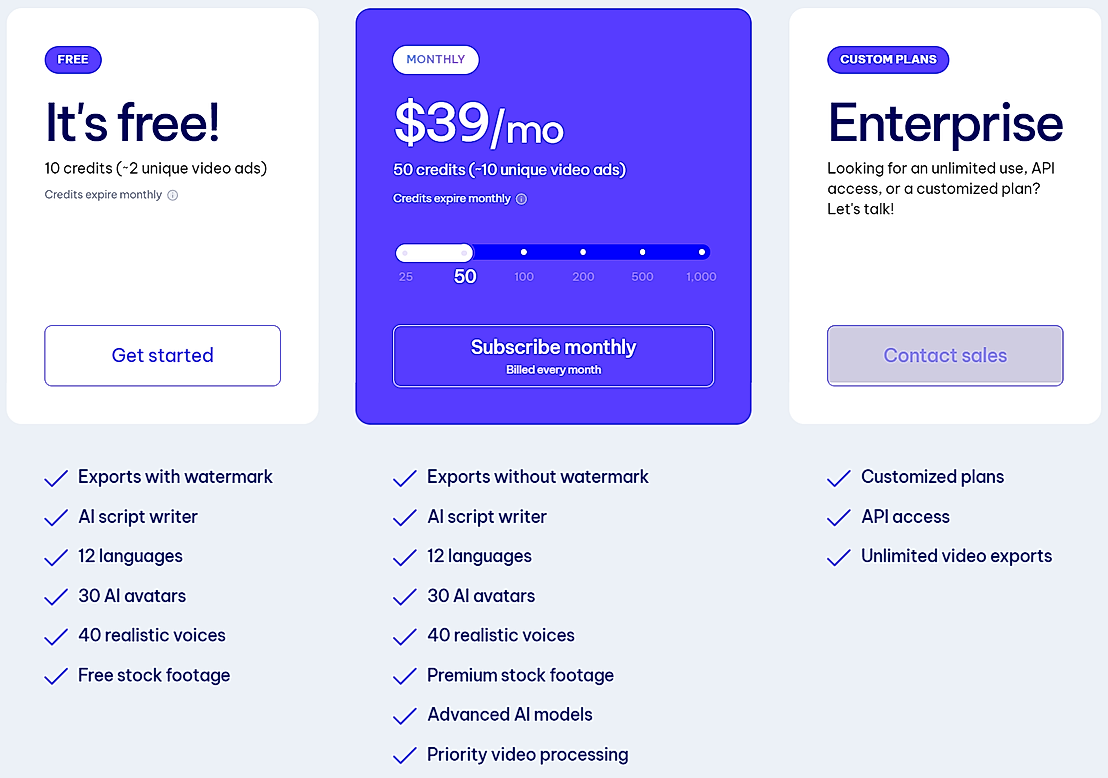The image depicts a webpage showcasing various subscription plans for a video ad creation service. The webpage is predominantly gray with accents in bright purple, and text in white and black.

The **first plan option** is labeled "Free":
- **Price:** Free
- **Credits:** 10 credits per month (expire monthly)
- **Unique Video Ads:** 2
- **Button:** Purple "Get Started"
- **Features:**
  - Exports with watermark
  - AI script writer
  - Available in 12 languages
  - Access to 30 AI avatars
  - 40 realistic voices
  - Free stock footage

The **second plan option** is titled "Monthly":
- **Price:** $39 per month
- **Credits:** 50 credits per month (expire monthly)
- **Unique Video Ads:** 10
- **Price Increment Chart:** $25, $50, $100, $200, $500, and $1000
- **Button:** Purple "Subscribe Monthly"
- **Billing:** Billed every month
- **Features:**
  - Exports without watermark
  - AI script writer
  - Available in 12 languages
  - Access to 30 AI avatars
  - 40 realistic voices
  - Premium stock footage
  - Advanced AI models
  - Priority video processing

The **custom plan option** is labeled "Enterprise":
- **Description:** Tailored for unlimited use, API access, or other customized needs. 
- **Button:** Contact Sales
- **Features:**
  - Customized plans
  - Full API access
  - Unlimited video exports

The page combines functionality with a clean aesthetic, ensuring the user can easily navigate and understand the different offerings.